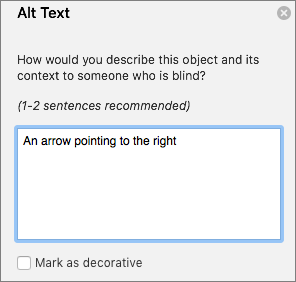This is an illustrative screenshot on a gray background featuring black text at the top that reads "Alt Text." Below it, there is a white rectangle outlined in thin blue, containing a right-pointing arrow. Beneath this rectangle, an unchecked white checkbox is labeled “Mark as decorative.” The entire image is framed by a thin black border with no photographic elements or depictions of people, animals, plants, buildings, or vehicles. The image is entirely textual.